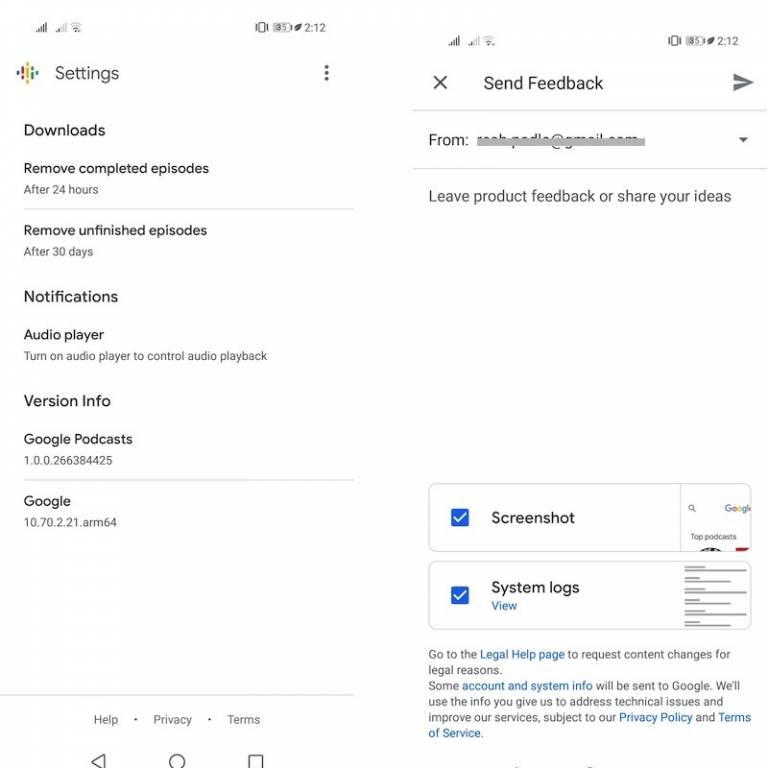This screenshot, taken at 2:12 PM, showcases a user's Google settings interface on a device with a white background. The visible settings include options for downloads, site feedback, screenshots, and system logs, among others. The device's status bar indicates a half-charged battery and a weak Wi-Fi signal, suggesting the user may be in a calm and relaxed environment.